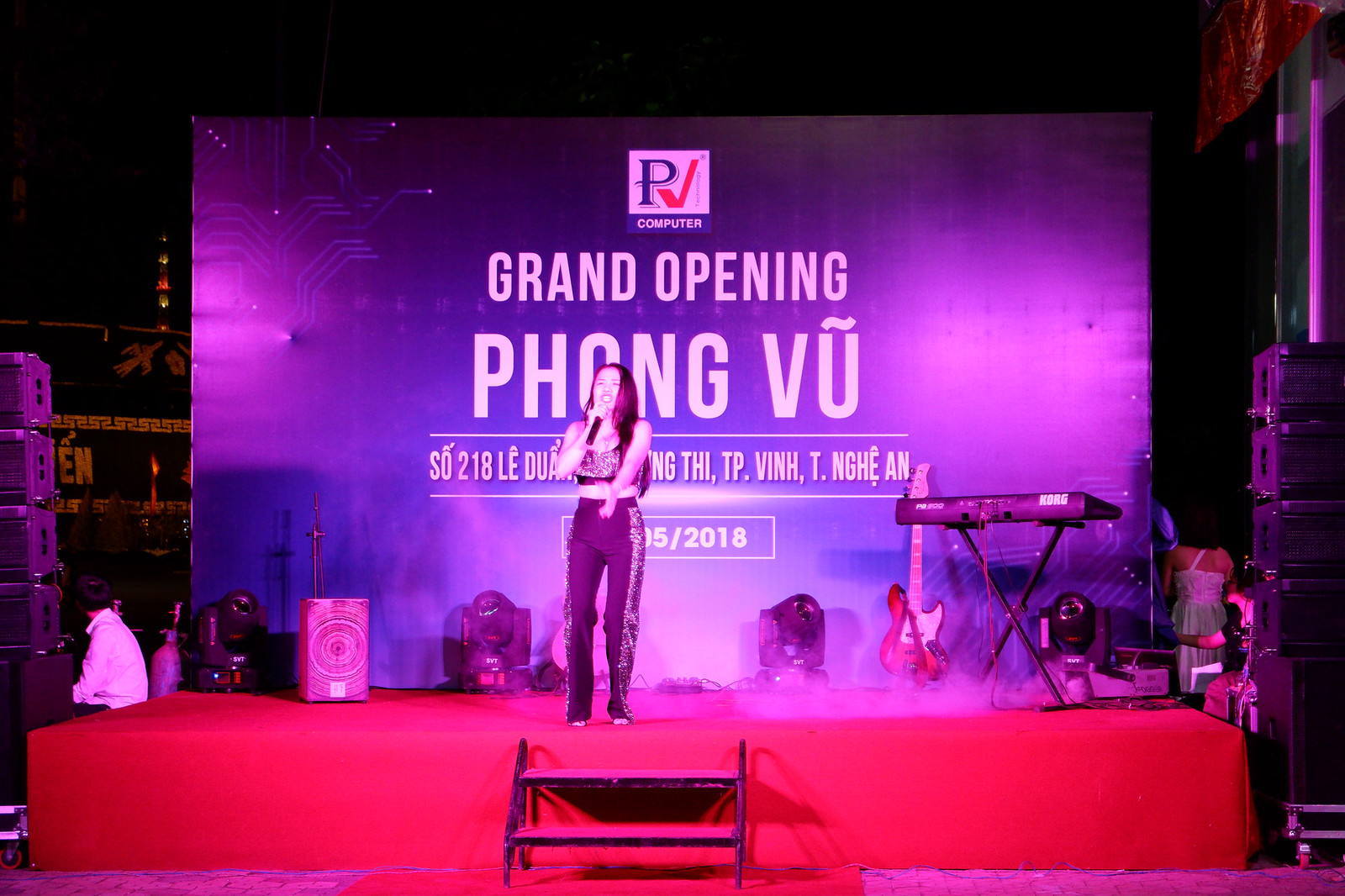The image captures an energetic moment during the grand opening of "Fong Vu," as an Asian woman, approximately 30-35 years old, takes center stage. She is dressed in stylish black pants with gold embellishments along the sides and a black, sequined tank top. Holding a microphone in her right hand, she appears to be performing or delivering a speech. The stage itself is vibrant with a red floor and two steps at the center, providing easy access. The backdrop prominently displays the text "Grand Opening Fong Vu" along with the PJ Computer logo at the top center. Musical equipment, including a keyboard to the right, an electric guitar leaning against the backdrop, and stacks of black speakers on both far edges, hint at a lively event atmosphere. Additionally, an address in a different language is visible, adding a touch of cultural specificity to the setting. The overall colorful image exudes excitement as lights illuminate the scene, making the grand opening event visually striking.